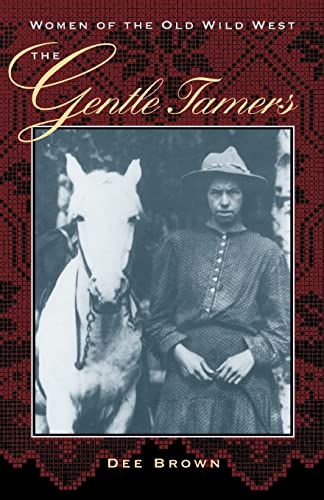This image resembles the cover of a book, displayed in a vertical rectangle format. The background features a design evocative of old-fashioned embroidery, with a blend of browns, reds, and black hues, reminiscent of needlepoint patterns. At the top, the title "Women of the Old Wild West" is prominently displayed in white text, followed by the subtitle "The Gentle Tamers" in cursive yellow lettering.

The centerpiece of the cover is a black-and-white photograph occupying a substantial portion of the space. On the right side of the photograph, a woman is depicted. She is dressed in pioneer-style clothing—a long-sleeved, button-down shirt, and a long skirt. Accessorized with a large sun hat, she stands with her hands clasped in front of her, exhibiting a stern demeanor with a slight frown. Beside her, on the left, stands a noble white horse, adorned with reins and a bridle, staring directly into the camera with its dark eyes.

At the bottom of the cover, the author's name, Dee Brown, is displayed, indicating their authorship of the book. The overall composition melds historical imagery and a nostalgic design, capturing the essence of the women who shaped the untamed landscapes of the Old Wild West.